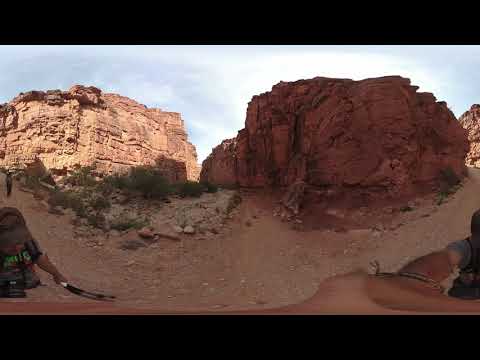In this detailed image, we see a person taking a video selfie in a rocky desert area, possibly in Arizona. The landscape features two massive rock formations; the one on the left is illuminated by the sun, appearing very light, while the one on the right is cast in shadow, giving it a dark red hue. The ground is dusty and gravelly, with a network of paths that extend left, right, and straight ahead. The valley-like terrain is partially shaded by the rock structures, with the sky above showing patches of blue mixed with white clouds, indicating a partly cloudy day. Additional details include sparse bushes nestled between the rocks and glimpses of another person (or possibly the same person seen in the selfie) either sitting or taking in the view. The composition suggests the photo might have been taken with a fisheye lens, adding a panoramic quality that captures the expansive, rugged environment.